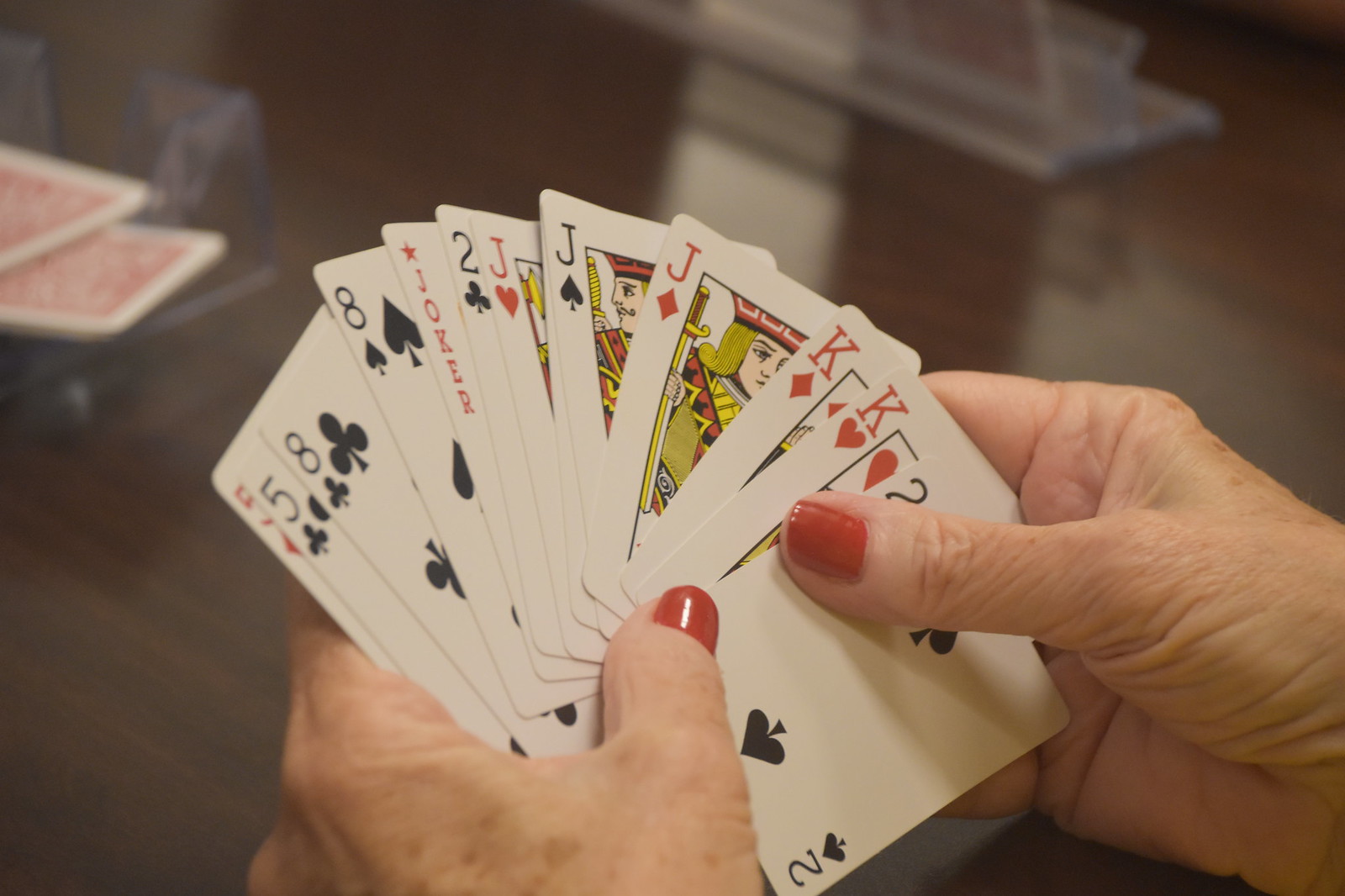In this detailed, up-close photograph, we focus on an elderly Caucasian woman's hands, distinguished by red fingernail polish adorning her well-groomed nails. Her skin, marked by the passage of time, features both wrinkles and brown liver spots, possibly interspersed with freckles. The woman grips a diverse array of playing cards with both hands, her thumbs prominently visible.

The foreground of the image is crystal clear, showcasing the intricate details of her cards, which include combinations of hearts, diamonds, clubs, and spades. Specifically, she holds a hand consisting of five red-suited cards, a five of clubs, eight of clubs, eight of spades, a joker, two of clubs, jack of hearts, two of spades, jack of diamonds, king of diamonds, king of hearts, and another two of spades. This varied collection suggests she may be engaged in a game of rummy, where forming pairs or groups is crucial. Notably, possession of another jack would significantly strengthen her hand.

The background, rendered in softer focus, reveals a brown table that spans beneath and beyond her hands. To the left of the image, a plastic tray holds several additional cards, while to the right, a card holder conceals an unspecified number of cards. This setup enhances the sense of a strategic, focused moment in the midst of a card game.